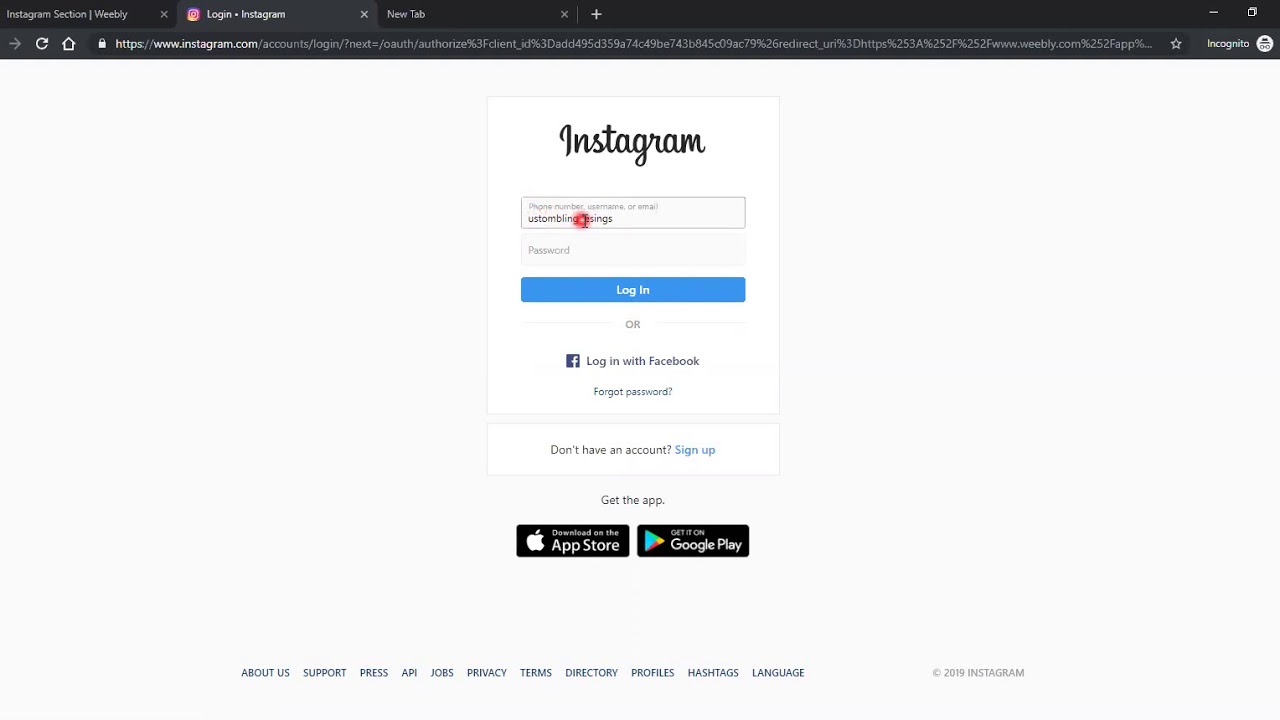The image showcases a browser window in incognito mode, displaying the Instagram login page. The browser has a black border at the top, containing three open tabs labeled: "Instagram Section – Weebly," "Login Instagram," and "New Tab." There is also a plus sign to add another tab. Just below the tabs, there is a series of navigation icons: an arrow pointing to the right for forward navigation, a circular arrow for refresh, and a home symbol. The URL bar shows the address "https://www.instagram.com/accounts/login/?next=/...," indicating it is the Instagram login page.

The background of the page is entirely white, with a prominent white rectangle in the center. At the top of this rectangle, "Instagram" is written in script font. Inside the main white rectangle, there's a smaller input field labeled "Phone number, username, or email" in gray text. A partially obscured input field appears below, filled with black dots for privacy with the letters "Sings" visible. Below this is another input field labeled "Password" in gray text. A blue button underneath reads "Log In" in white text, followed by an option to "Log in with Facebook." At the bottom of the white rectangle, it says "Forgot password?" indicating a link for users to recover their login details.